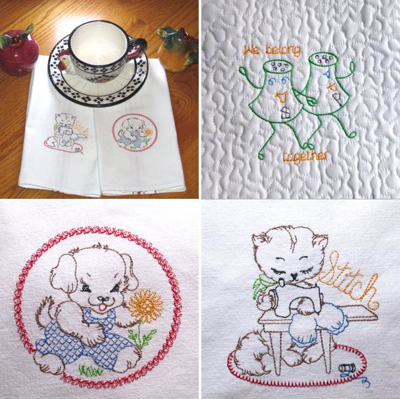The image is a composite of four photos arranged into a mosaic, forming a larger square. In the upper left quadrant, a teacup with a black and white patterned saucer rests on top of two embroidered linen cloths. Surrounding the teacup are a few knickknacks, including objects resembling an apple and a crocodile. The upper right quadrant showcases another embroidered linen featuring a whimsical design of a salt shaker and a pepper shaker holding hands and walking together, accompanied by the text "We belong together." In the bottom left quadrant, there is an intricate embroidery of a dog wearing overalls and playing with a sunflower. The bottom right quadrant displays an embroidered cat operating a sewing machine, working on a piece of fabric. The linens are primarily white but feature vibrant accents of pink, green, orange, and blue, bringing the detailed and charming designs to life.